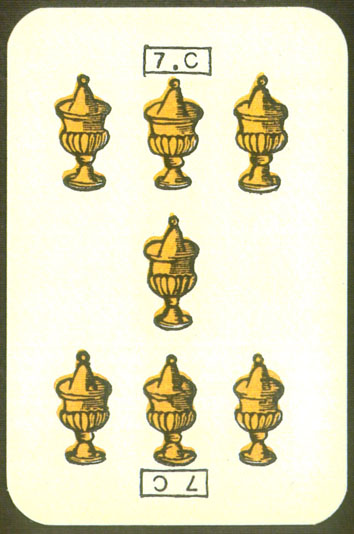This image displays a meticulously hand-drawn playing card. The card is rectangular with rounded edges and features a dark brown border. The card itself has a yellowish-white hue, with varying shades that give it an aged appearance. 

At both the top and bottom, small hand-drawn gray rectangles house gray lettering, with "7.C" at the top and the inverted "7NC" at the bottom. The central design includes seven gold chalices—three aligned in the top row, one in the center, and three in the bottom row. Each chalice is outlined with dark gray pencil markings and filled with an uneven, slightly outside-the-lines application of smooth gold coloring.

The chalices boast a detailed design, with a lid, an ornate base, and a long, rounded stem. While all the chalices share the same basic structure, each one is sketched with subtle differences, adding unique characteristics to the design. The overall look of the card combines historical elegance with the charm of hand-drawn art.